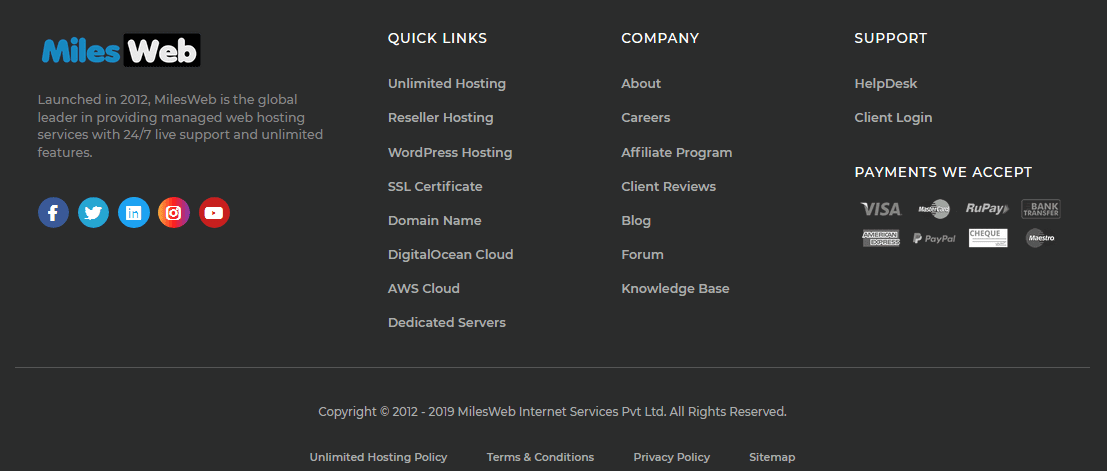This image showcases the branding and informational overview of Miles Webb, a company established in 2012 that specializes in managed web hosting services. The image features an entirely black background. The company name, "Miles Webb," is displayed prominently with "Miles" in blue and "Webb" in white. The text "Webb" is set against a black square background, enhancing its visibility.

Miles Webb is recognized as a global leader in providing managed web hosting services, featuring 24/7 live support and unlimited features. Social media icons on the image indicate the company can be found on Facebook, Twitter (X), Instagram, Indeed, and also via email, denoted by a circular icon with a white envelope.

The image lists several quick links for easy navigation, including options for Unlimited Hosting, Reseller Hosting, WordPress services, SSL Certificates, Domain Names, Digital Ocean Cloud services, AWS Cloud services, and Dedicated Services.

Additional clickable sections provide further information about the company, its career opportunities, affiliate programs, client reviews, blog, forums, and knowledge base. For customer support, there is a Help Desk and Client Login section.

The image also highlights various payment methods accepted by Miles Webb, such as Visa, RuPay, MasterCard, PayPal, American Express, and bank transfer. The copyright notice on the image states "2012 to 2019," and mentions their Unlimited Hosting Policy, Terms and Conditions, Privacy Policy, and Sitemap, indicating a comprehensive range of services and information available on their website.